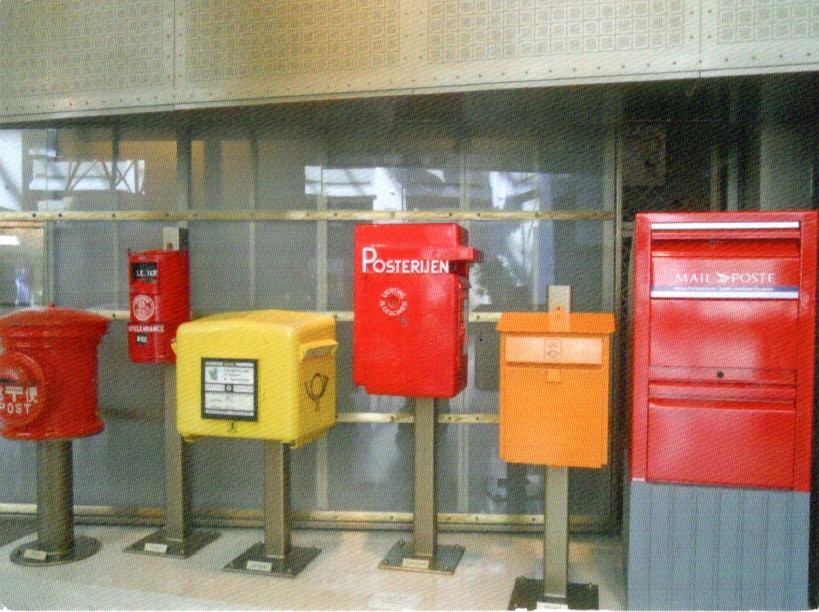This image depicts a series of six distinct postboxes arranged outside an industrial-looking building with a metallic, square-patterned facade and an overhang partially covering them. The photograph appears to be old and grainy, possibly taken on film. The postboxes are aligned, with the four on the left mounted on metal stands and small placards at their bases. From left to right:

1. The far-left box is red and cylindrical, resembling a fire hydrant, labeled "POST."
2. To its right is a smaller, similarly cylindrical, bright red mailbox.
3. Next, a bright yellow, square-shaped box features a white square on its front for mail type identification.
4. Following this is a reddish rectangular box marked "POSTERIJEN," with a circular symbol underneath.
5. An orange, rectangular mailbox is situated to the right of the "POSTERIJEN" box and lacks visible text.
6. The final and largest box on the right is bright red, positioned atop a silverish platform, and marked "MAILPOST" and "POSTE."

This assortment of postboxes suggests potential international origins, indicated by the varied labels and styles, making it a compelling display of postal history.